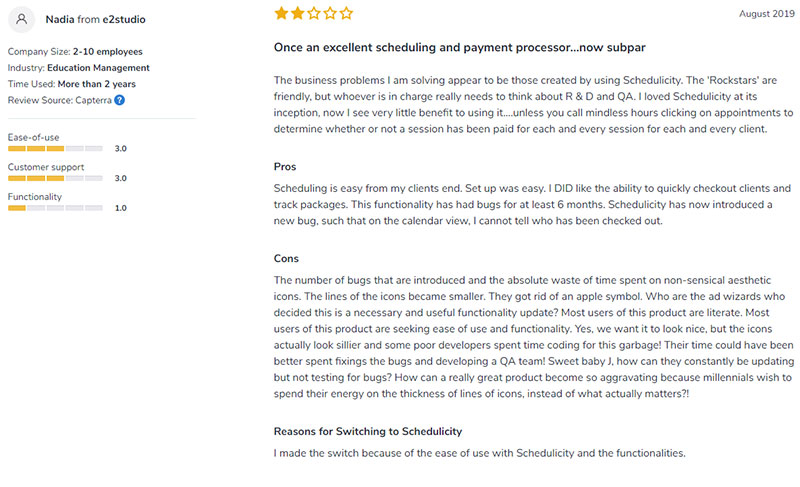Here is a detailed and cleaned-up descriptive caption for the image:

---

📉 **User Review: Schedulicity** 📉

⭐️⭐️☆☆☆ (2/5 Stars)  
📅 August 2019

**Title:** Once an Excellent Scheduling and Payment Processor, Now Subpar

**Review:** 

Previously a stellar platform, Schedulicity has recently declined in quality. The application, once praised for its excellent scheduling and payment processing capabilities, now presents more problems than solutions. The constant issues appear to be generated by the use of Schedulicity itself. 

Although the customer service team, referred to as 'rock stars,' is friendly, the leadership seems to lack focus on Research and Development (R&D) and Quality Assurance (QA). At its inception, the app was highly beneficial, but currently, it offers limited advantages. The most significant issue is the cumbersome process of manually verifying whether each session for every client has been paid, contributing to countless hours of mindless clicking on appointments.

**Pros:** 
- User-friendly scheduling interface for clients
- Easy setup process
- Ability to quickly check out clients and track packages

**Cons:**
- Persistent functionality bugs for over six months
- New bugs impairing calendar view functionality, making it unclear who has been checked out
- Waste of time due to frequently introduced, non-essential icons

---